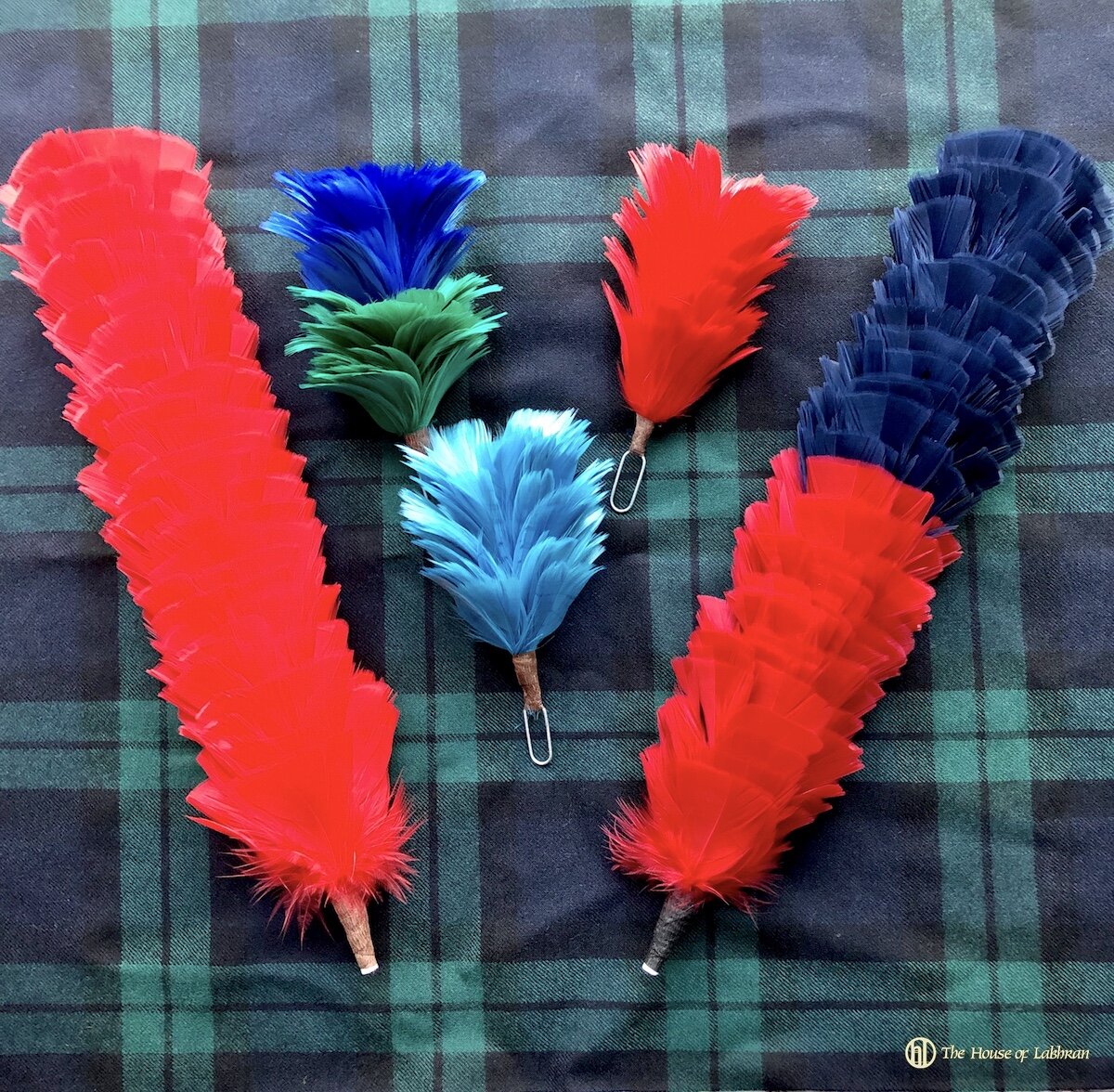The photograph features a checkered tartan fabric background in shades of green, navy blue, black, and teal. At the bottom right corner, there is yellow text that reads "The House of London" along with a small logo. Five feather dusters are arranged on the fabric. On the left, a tall, solid red feather duster with a brown base stands out. To its right is another large feather duster with a navy blue top and a red bottom. Further to the right are three smaller feather dusters: one solid red, one light baby blue, and one with a dark blue top and a dark green bottom. All the feather dusters are neatly placed on the plaid background, creating an interesting contrast of colors and textures.